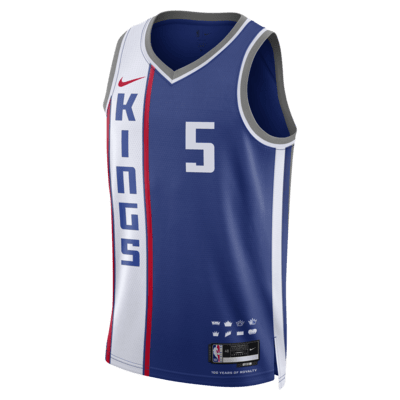The image showcases a men's sleeveless basketball jersey prominently featuring the colors blue, white, and red. The jersey's primary color is blue, which covers the majority of the right side, stretching across to the center and partially towards the left. A distinctive red stripe runs vertically from the top to the bottom alongside this blue section. The neckline is a V-neck outlined in gray with an additional white trim around it, matching the gray armholes.

On the blue chest area of the jersey, the number '5' is boldly printed in white. Adjacent to this, on the left side, the text 'KINGS' is written vertically in white on a stripe bordered by red lines. Above this text, the red Nike swoosh is clearly visible. A white stripe flows down the left side of the jersey. Near the bottom left corner, there is a label, which includes the NBA logo and some manufacturing information.

The background of the image is plain, ensuring that the jersey remains the focal point. The design includes various elements like multiple Kings logos above the NBA emblem, adding to its detailed and elegant appearance.